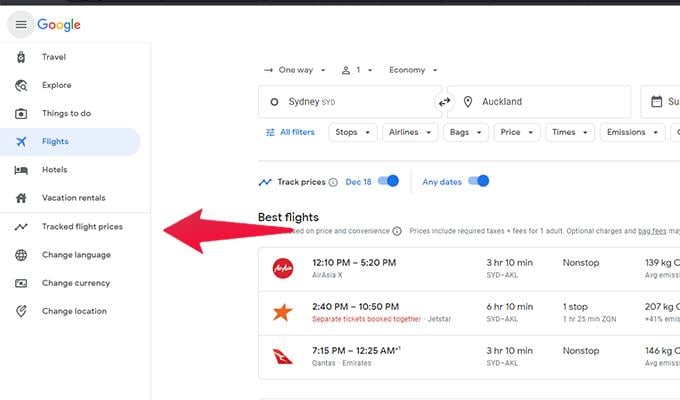The top left corner of the image features a hamburger menu alongside the Google logo. Below this is a column displaying options such as Travel, Explore Things to Do, and Flights. This is likely a travel search interface given options like "change language," "change currency," and "change location."

A prominent red arrow points to the left, guiding attention towards a runway image with a person labeled "economy, Sydney." Further down, an "all filters" section enables users to filter flight options by stops, airlines, bags, price, and time. There's also a "check prices" button set for December 18, with an 80-day lookahead toggle for finding the best flights based on price and convenience, including required taxes and post fees for one adult and optional charges for back payments.

Another segment highlights a flight option in a red circle, departing at 12:00 PM and arriving at 5:20 PM via Air HX, with a flight duration of 3 hours and 10 minutes. Additional flight details mention no stops, 138kg luggage limit, and an alternative flight from 2:40 PM to 10:50 PM.

Summary information includes separate tickets booked together for a total travel time of 6 hours and 10 minutes, with an initial stop of 1 hour and 24 minutes. The last segment notes a return leg from 10:50 PM to 12:25 AM, with quantities set to 3 hours and 10 minutes, no stops, and a 146kg luggage limit.

Overall, the image encapsulates a comprehensive flight search interface complete with various filters, travel details, and price comparisons for flights to Sydney.